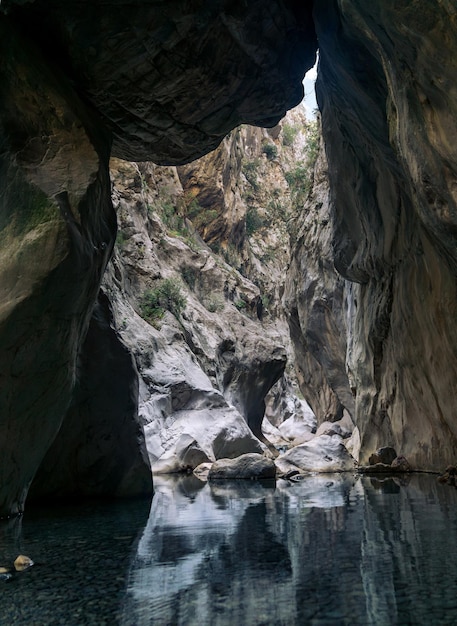The image showcases a serene, cavernous scene dominated by a mesmerizing body of water within a large cave. The cave walls, composed of jagged gray and brown rocks, create a rugged enclosure. Green trees and plants grow sporadically on the walls, adding a touch of life to the otherwise stark environment. The water, clear and still like glass, perfectly reflects the rocky walls above, casting shadows that enhance the cave's mysterious allure. The water appears shallow, allowing visibility of the rocky bottom and various stones jutting out from its surface. In the center of the image, light filters down through a skylight opening high above, revealing a sliver of sky and suggesting an external world beyond the cavern. On the left side of the picture, there seems to be another potential entrance to the cave, marked by a rock ledge precariously teetering on the edge. This tranquil, otherworldly scene captures the hidden beauty and intricate details of the subterranean environment.